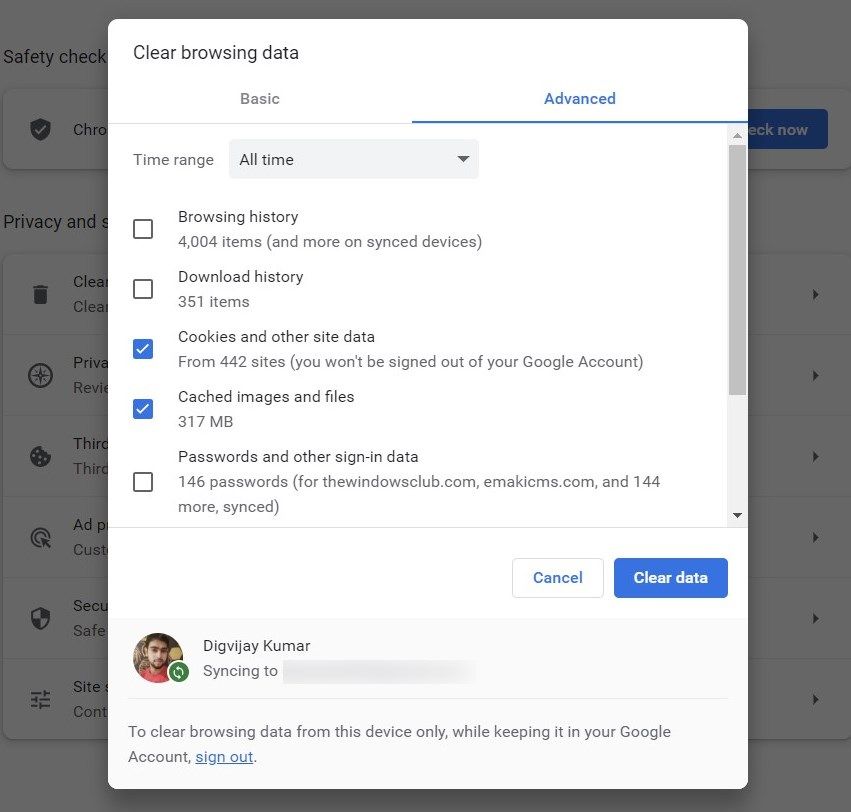The image displays a screenshot of the Google Chrome settings interface, specifically highlighting the "Clear browsing data" pop-up window. The window is open to the "Advanced" tab, indicated by the pressed "Advanced" option on the right, as opposed to the unselected "Basic" option on the left. At the top, the pop-up includes a "Time range" dropdown menu set to "All time."

Below the dropdown menu, there are five checkboxes aligned vertically on the left side. The status of these checkboxes is:
1. "Browsing history" – unchecked
2. "Download history" – unchecked
3. "Cookies and other site data" – checked
4. "Cached images and files" – checked
5. "Passwords and other sign-in data" – unchecked

On the right side of the screen are two buttons: "Cancel" on the left and "Clear data" on the right. Additionally, the profile section at the top right corner displays a profile icon with the name "Digvijay Kumar" next to it, followed by the text "Syncing to" and a blurred-out rectangle.